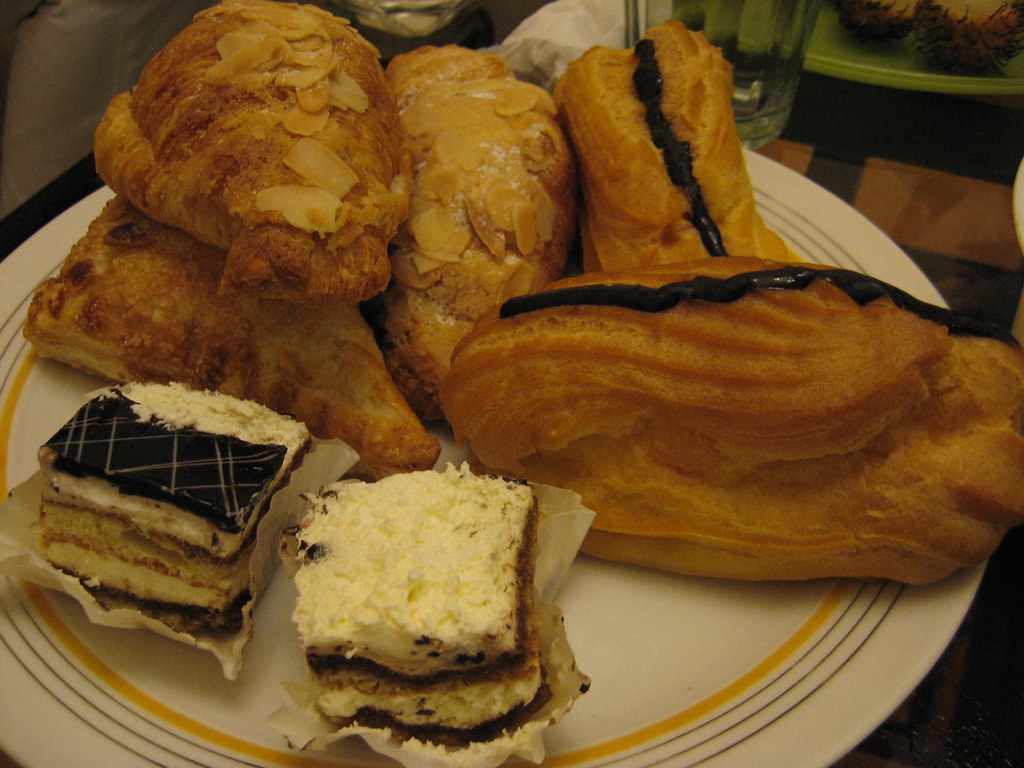This photograph captures a delectable assortment of dessert pastries artfully arranged on a white ceramic plate with intricate concentric circles—yellow on the inner ring and three brown rings on the outer edges. The plate boasts a delightful variety of treats. In the lower left, several square-cut cakes, possibly tiramisu, rest inside ridged cupcake papers, with multiple layers and a dollop of frosting crowning each one. Dominating the center, there are two cream puffs adorned with stripes of chocolate frosting, while nearby, unfamiliar pastries with a pulpous texture and a dusting of shredded nuts offer a visual and gustatory contrast. Additionally, two almond-covered pastries and a turnover—likely filled with apple or cherry—complete the tantalizing spread. The photo's composition is enriched by the surrounding elements: a person in white pants enters the frame from the top left corner, a glass cup and a tantalizing glimpse of another dessert-laden green plate appear in the top right. The lighting is soft and orange, casting a warm, inviting glow over the delectable scene.